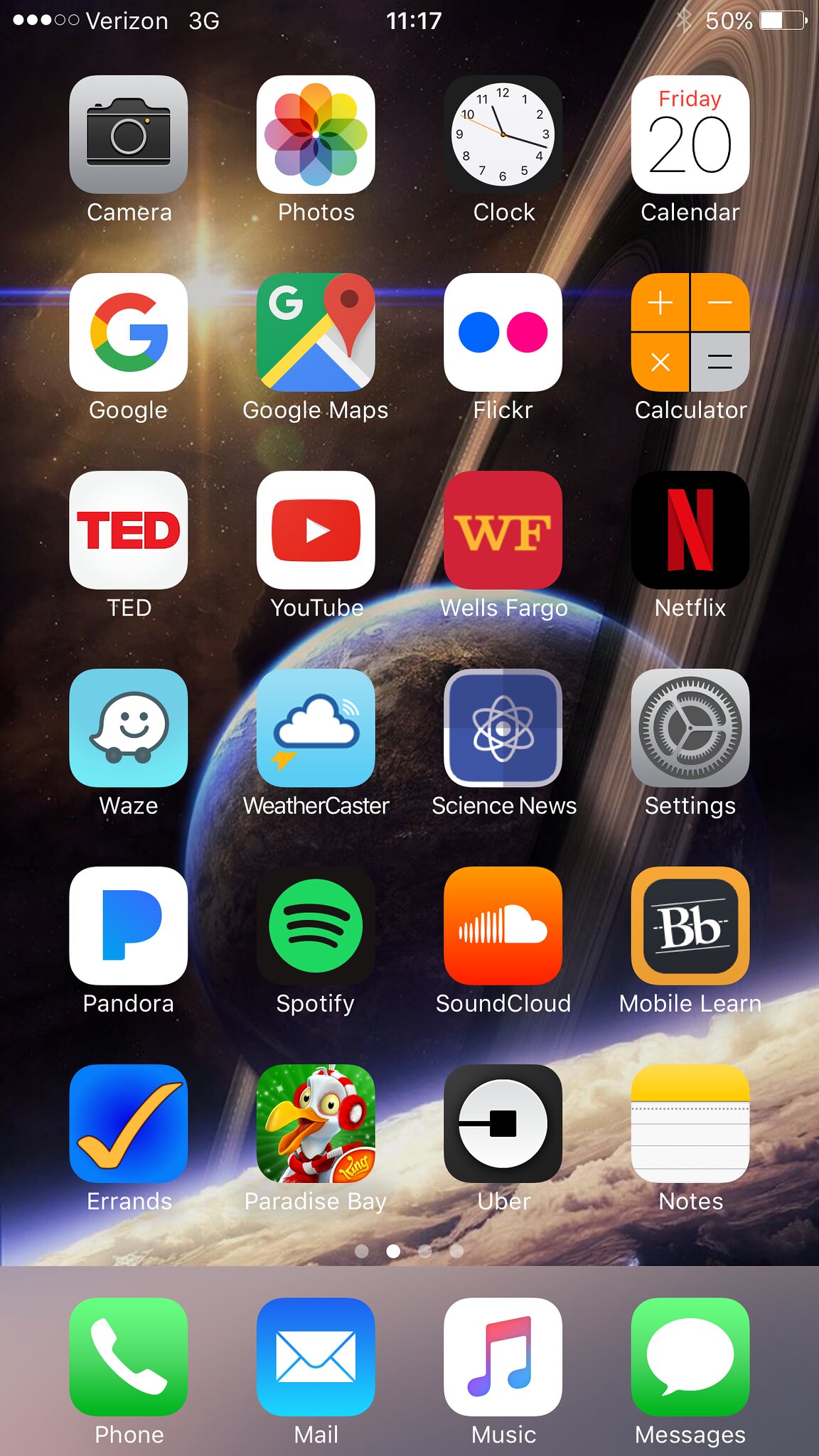This is a detailed screenshot of an iPhone's home screen displaying a diverse array of applications and a unique space-themed background. 

The status bar at the top shows the device is connected to Verizon 3G with three bars of signal strength, the time is 11:17, and the battery level is at 50%. The main home screen features multiple rows of app icons arranged neatly:

1. At the top row, we find the Camera, Photos, Clock, and Calendar apps.
2. The second row includes Google, Google Maps, Flickr, and Calculator.
3. The third row contains TED, YouTube, Wells Fargo, and Netflix.
4. The fourth row has Waze, Weather, Caster, Science News, and Settings.
5. The next row displays Pandora, Spotify, SoundCloud, and Mobile Learn.
6. Below that, there are icons for Errands, Paradise Bay, Uber, and Notes.

The main dock at the bottom houses the Phone, Mail, Music, and Messages apps.

The background wallpaper is an imaginative depiction of an Earth-like planet adorned with a set of Saturn-like rings, with a star gleaming behind it. The scene is further dramatized by clouds or possibly dust clouds, creating an ethereal and fantastical outer space ambiance. The perspective suggests a view from another planet with an atmosphere, though it is scientifically improbable.